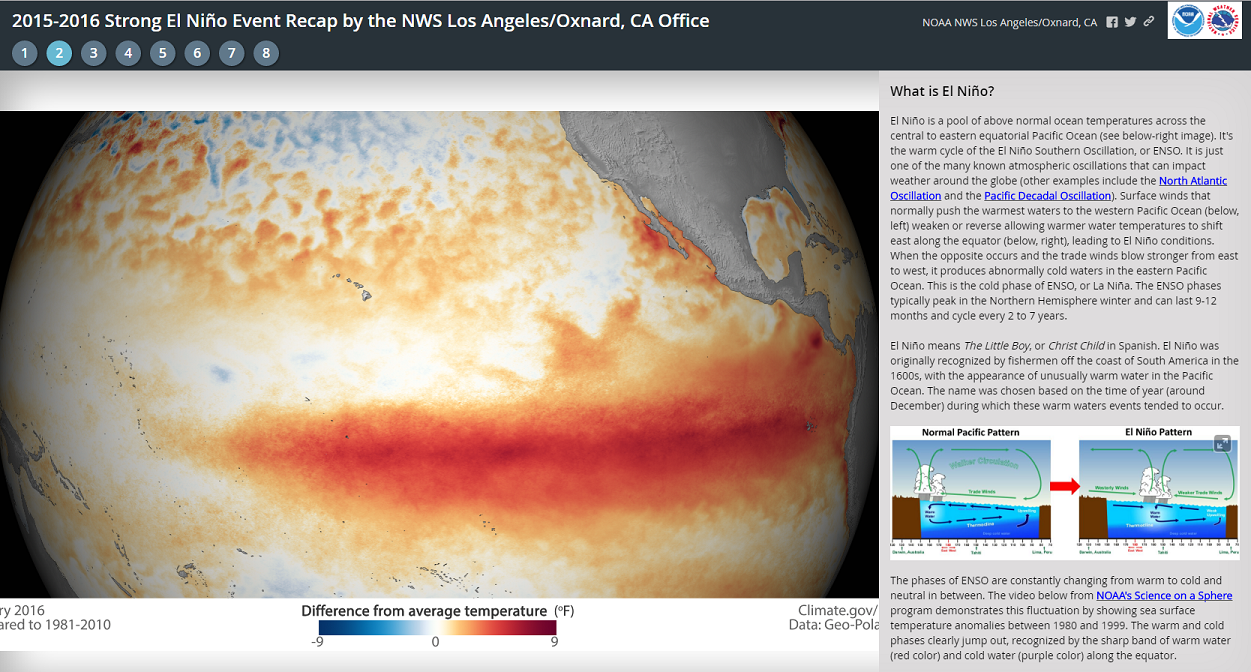**Descriptive Caption:**

We are viewing a detailed image of a webpage recapping the 2015 to 2016 strong El Niño event, as presented by the NWS Los Angeles—Oxnard, California office. The top border features a black background with the title in white text: "2015 to 2016 Strong El Niño Event Recapped by the NWS Los Angeles—Oxnard California Office." Below this are gray circles numbered one to eight, with the number two highlighted in blue. In the upper right-hand corner, there is white text that reads "NOAA NWS Los Angeles—Oxnard California," followed by icons for Facebook and Twitter, and a white chain link symbol. 

On the right, a white box contains two logos: a blue round one and another with orange text. To the left, the page displays a thermal heat image of Earth, showing parts of the United States, Mexico, and Central America. The ocean is depicted with various colors, highlighted by a rich orange band along the equator, indicating significant temperature variations. 

A legend at the bottom, partially cut off, indicates that the image compares temperatures from 2016 to averages from 1981 to 2010. It provides a color scale from dark blue (negative nine degrees Fahrenheit) to deep red (positive nine degrees Fahrenheit). Additional text on the image mentions "climate.gov" before being cut off.

To the right, in a gray box with black text, there is an explanation of El Niño. It describes El Niño as a phenomenon characterized by above-normal ocean temperatures across the central to eastern equatorial Pacific Ocean, caused by weakened or reversed surface winds. The opposite phase, La Niña, involves stronger trade winds producing abnormally cold waters. The ENSO phases peak in the northern hemisphere winter and typically last nine to twelve months, cycling every two to seven years. The term "El Niño," meaning "little boy" or "Christ child" in Spanish, originated from South American fishermen in the 1600s.

Additionally, there's a labeled graphic contrasting the normal Pacific pattern with the El Niño pattern, using green and red arrows to denote water movements. The bottom of the page discusses how the phases of ENSO cycle between warm, cold, and neutral states, with a highlighted link to a NOAA Science on a Sphere program that demonstrates these fluctuations from 1980 to 1999 through sea surface temperature anomalies.